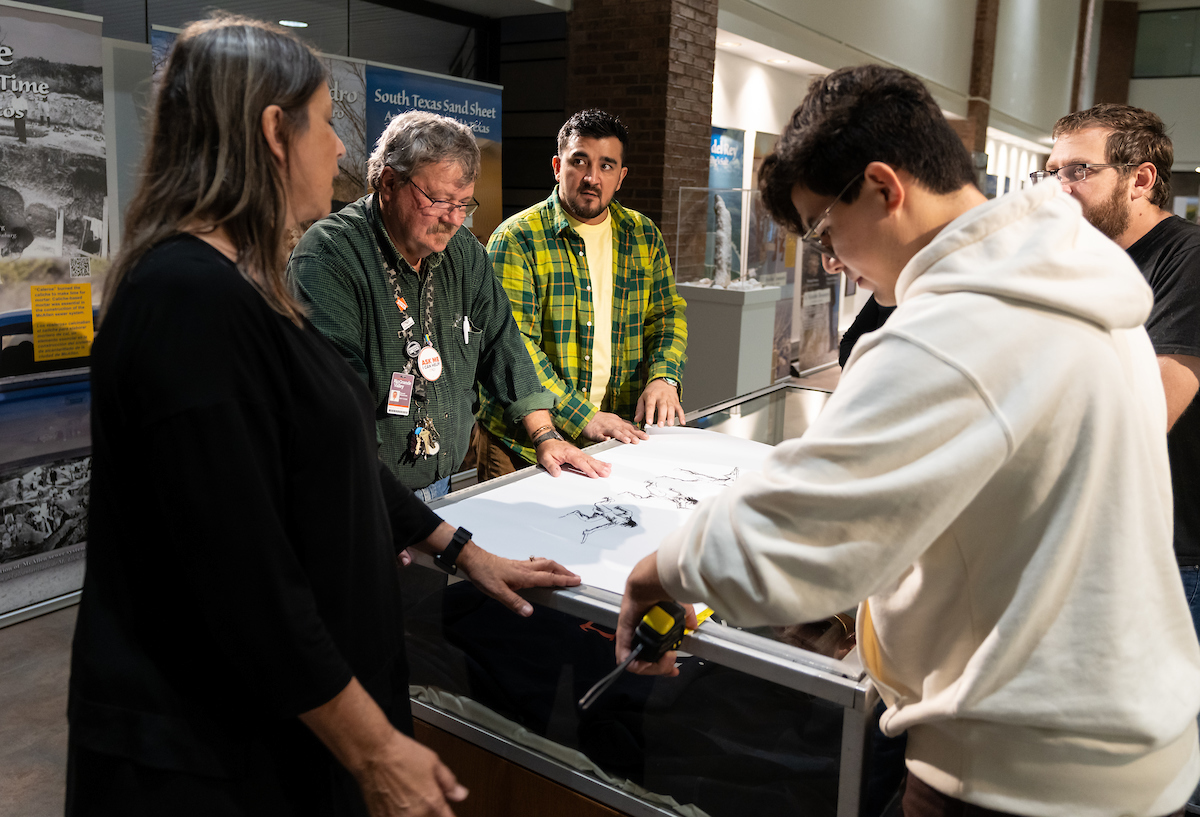In this detailed image inside a natural history museum, a group of five people appears to be engaged in a collaborative meeting around a glass-encased exhibit. The exhibit seems to center around the "South Texas Sand Sheet," as indicated by a sign in the background. The focal point of the group is a brown-haired woman in black, positioned on the far left yet centrally involved with the display, as her hand rests on the glass case. Surrounding her are four men of varying ages: one in a buttoned-down green shirt, one in an unbuttoned green flannel shirt, another in a white hoodie, and the last in a black t-shirt. Notably, three of the men are wearing glasses. They all seem focused on a paper drawing or design that is rolled out on top of the glass case, suggesting they might be preparing or discussing the details of the exhibit involving different types of sand. The man in the white hoodie is holding a ruler, seemingly taking measurements. The backdrop features a stand-up glass box and various images, indicating the room is rich with exhibits, contributing to the scholarly environment.